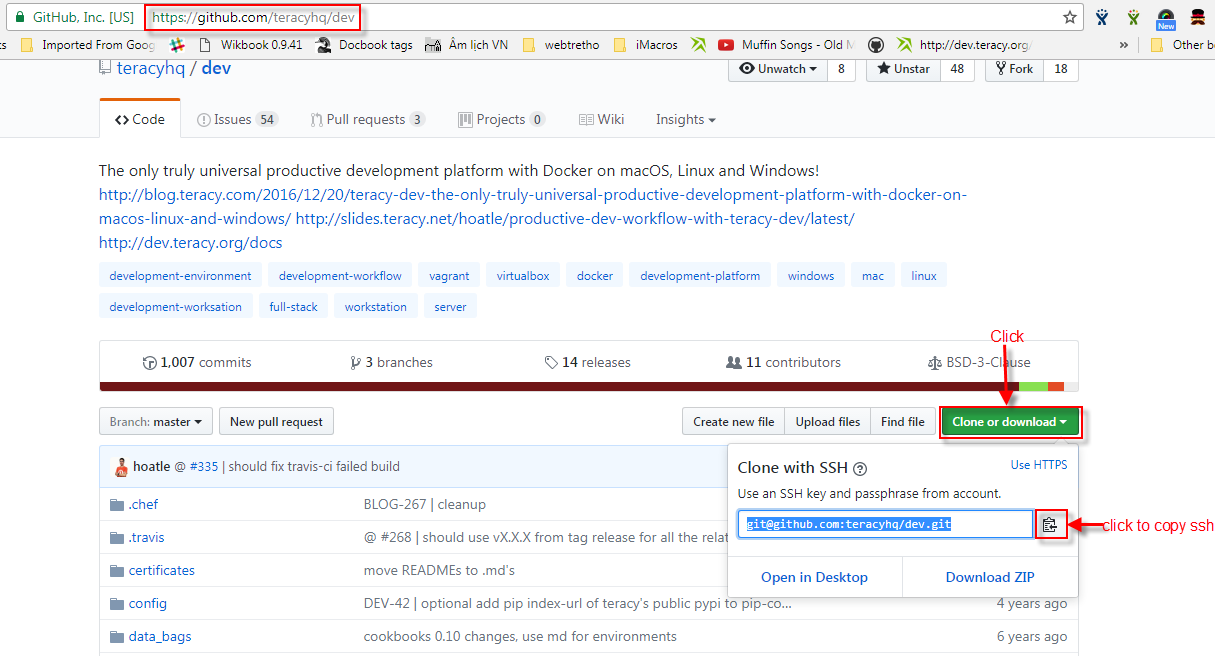This image displays a screenshot of a GitHub repository page from the website github.com, specifically from the repository located at "https://github.com/TerraSiteQueue/dev." The URL is highlighted with a red rectangle. At the top navigation bar of the repository page, there are tabs for 'Code,' 'Issues' with a count of 54, 'Pull Requests' with a count of 3, 'Projects' with a count of 0, 'Wiki,' and 'Insights.'

Below the navigation, a descriptive text reads: "The only truly universal productive development platform with Docker on Mac OS, Linux, and Windows." This is followed by a series of clickable blue links.

Further down the page, repository statistics are visibly noted: "1,007 commits, 3 branches, 14 releases, and 11 contributors." 

On the right-hand side of the page, there is a section titled "Clone or download," highlighted with an inserted annotation that includes a red arrow pointing down and the word "click" within the annotation. There's also an adjacent area marked as "Click to copy SSH."